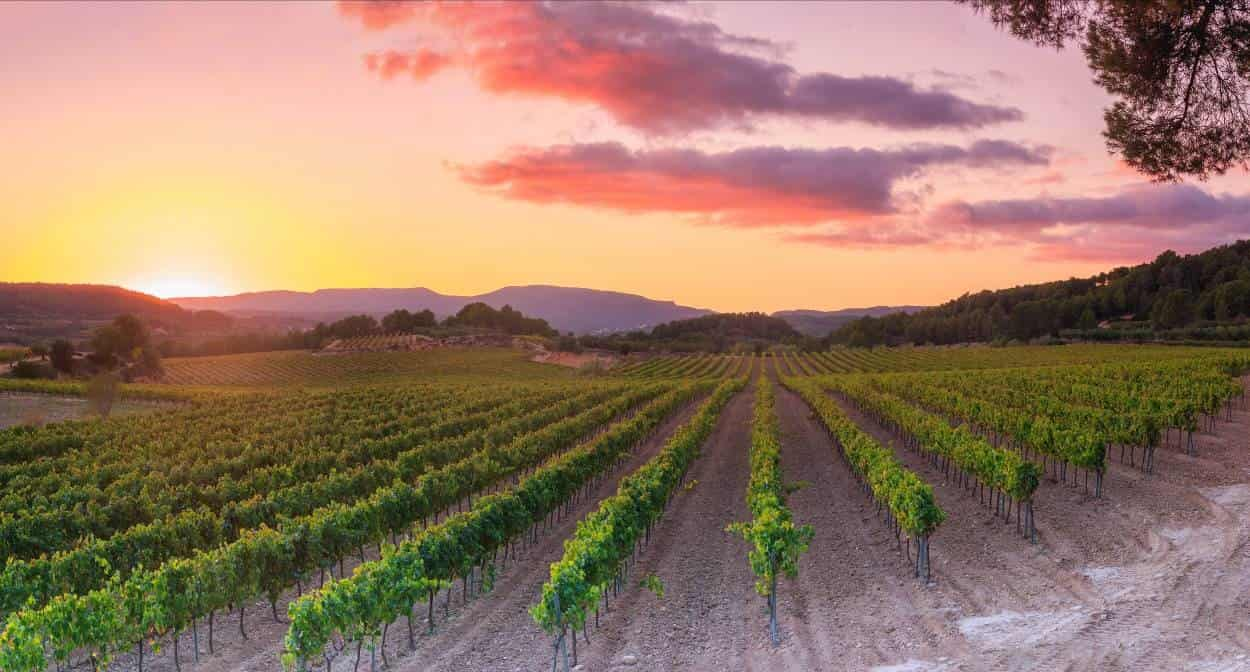In this picturesque vineyard scene taken at dusk, rows upon rows of grapevines neatly tied to two-foot poles stretch across the field, creating a striking pattern of green leaves interspersed with dirt walkways. The grapevines extend into the distance, under a sky transitioning from soft blue to a warm orange hue as the sun sets. On the left side, the sun dips behind a silhouetted mountain range, casting a serene glow over the vineyard. The sky above features pink and purple clouds, adding a splash of color to the tranquil scene. Bordering the vineyard, tall trees form a forest-like backdrop, framing the idyllic landscape.